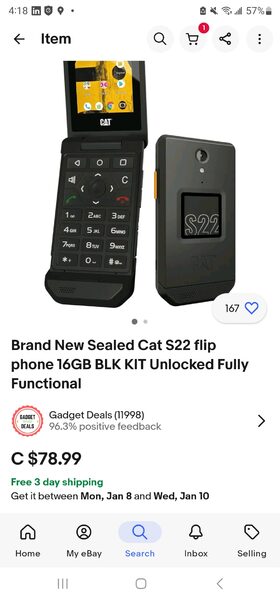The screenshot showcases a black flip phone, identified as a Cat S22 model, which appears to be an Android device. The phone is displayed on a plain white background, suggesting that the image might have been taken from an Amazon listing. The device features an old-school numeric keypad and is described as brand new and sealed. It has 16 gigabytes of storage and is unlocked, making it compatible with various carriers. The listing highlights it as a "fully functional gadget," priced at $78.99 with free three-day shipping offered at the bottom of the page. 

Additionally, the interface indicates that this is the first of two images available for viewing, as denoted by the two-dot image navigation indicator at the bottom. The store's navigation section is visible but does not seem familiar. The overall presentation is prominently focused on the phone against the simplistic white backdrop.